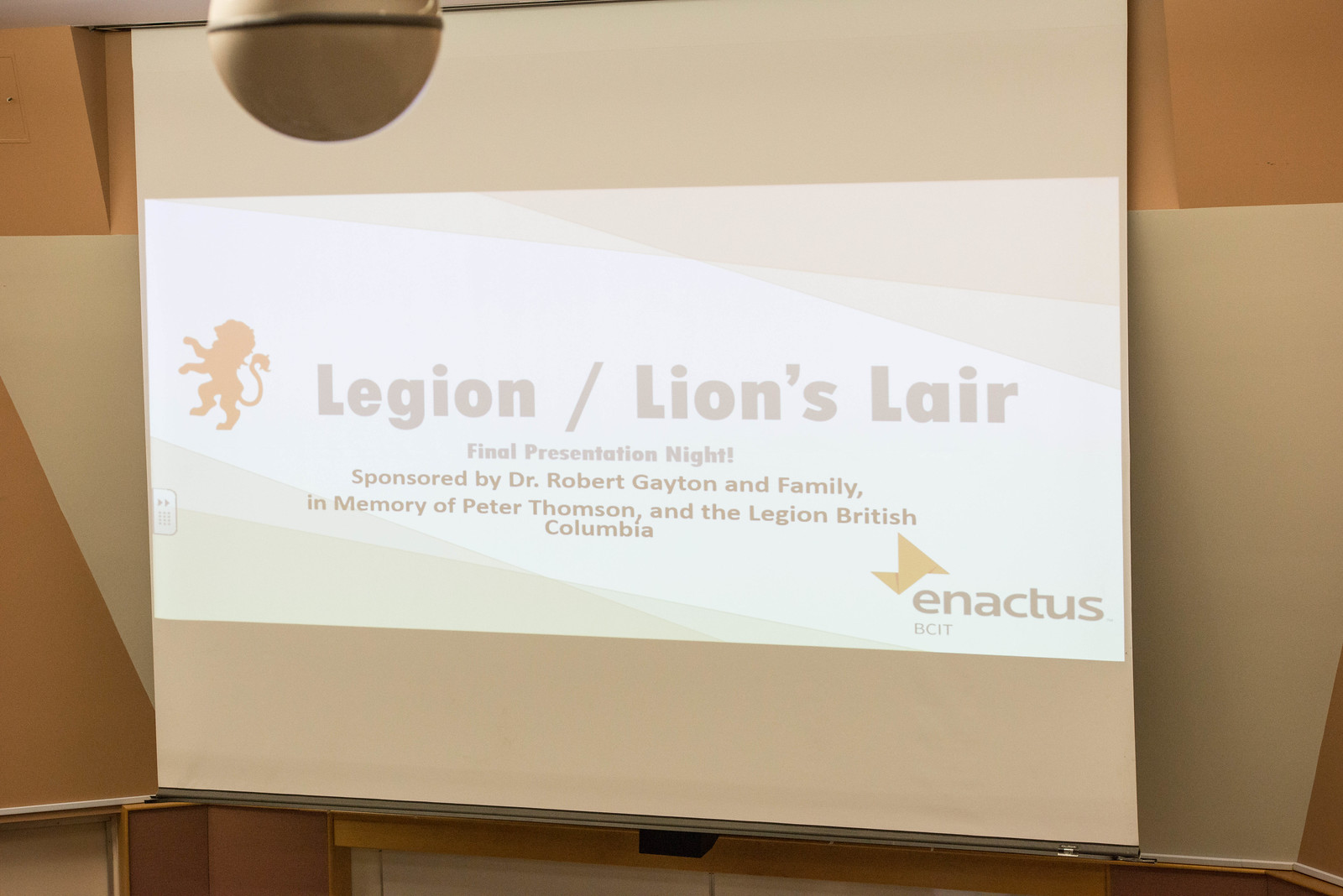The photograph depicts an indoor scene, likely set in a college auditorium or lecture hall. The focal point is a large projector screen mounted high up, with a whiteboard positioned beneath it. The screen displays a slide that features an orange silhouette of a lion standing upright on its hind legs, positioned on the left side. To the right of the lion, in large gray font, the text reads “Legion / Lions Lair.” Underneath, in smaller font, it continues with “Final Presentation Night, sponsored by Dr. Robert Gayton and family, in memory of Peter Thompson and the Legion British Columbia.” In the bottom right corner of the slide, there is an Enactus logo, accompanied by the acronym BCIT. The surrounding beige walls are angular and slanted, leading up to the ceiling, with the light from the projector spilling onto them. This setting suggests a formal presentation, possibly an academic or professional event.